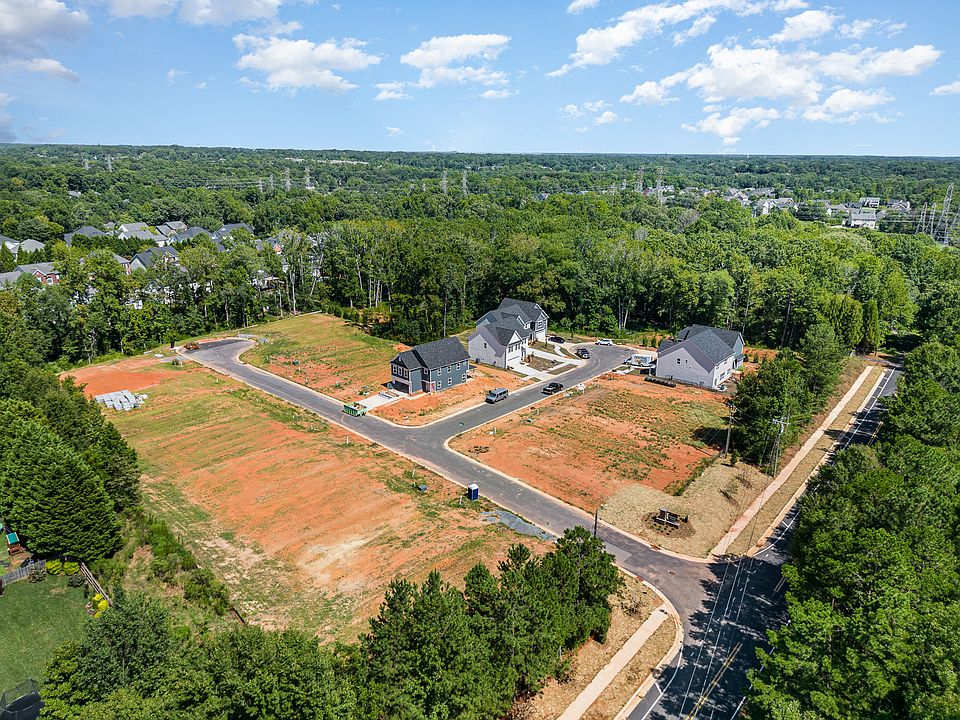The drone footage captures a suburban neighborhood development nestled within a lush, tree-filled area under a clear blue sky. Four newly constructed light gray homes with darker gray rooftops stand prominently on cleared patches of land, surrounded by tall green trees and red clay-like soil. The subdivision's layout is defined by paved asphalt roads winding through the area, while power lines can be seen in the distance. The scene reflects a mix of natural greenery and ongoing development, with some lots still awaiting construction.